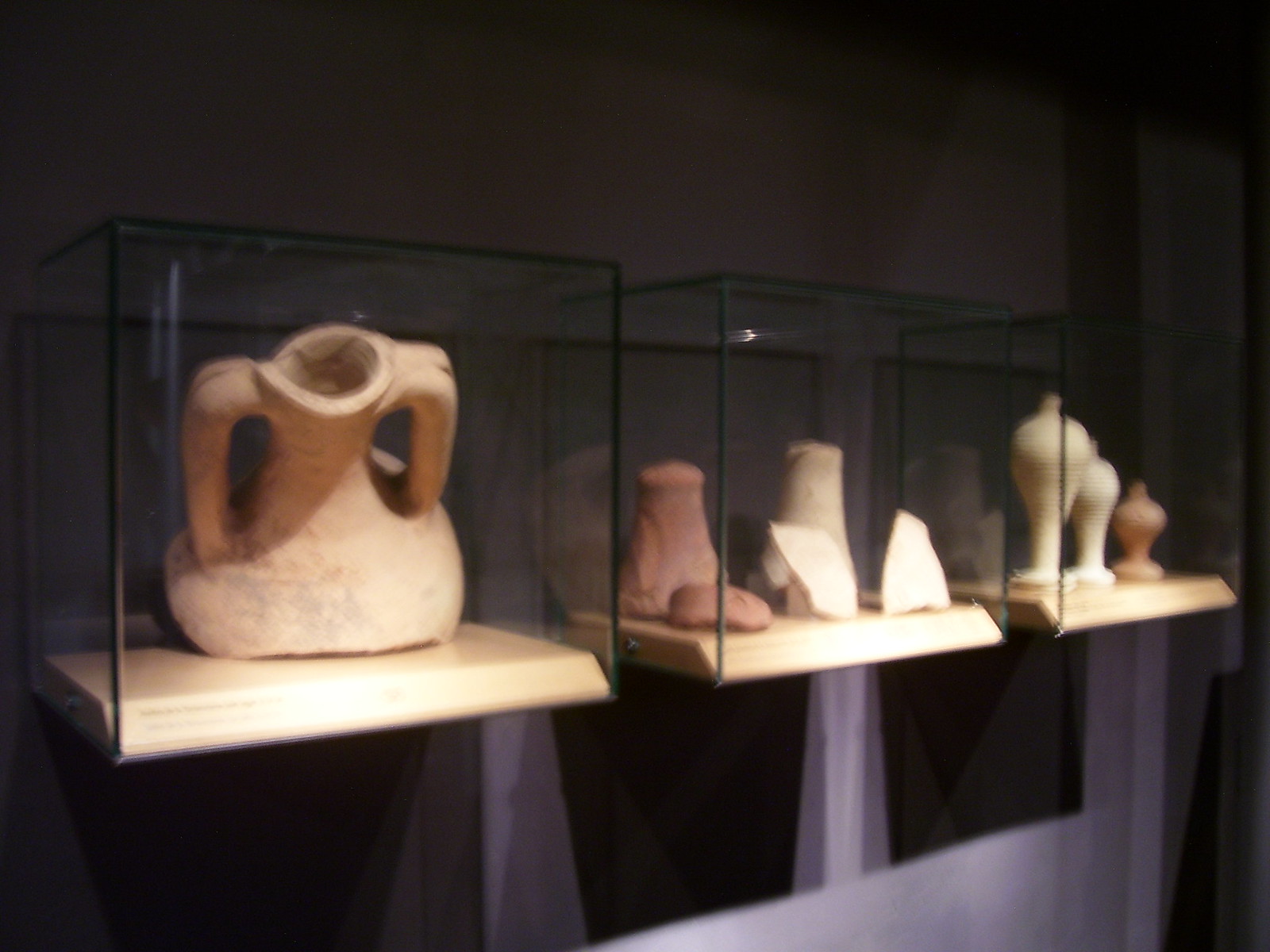The image captures a museum exhibit featuring three large glass cases mounted on a dark gray wall, each containing ancient pottery artifacts. The lighting is typical of a museum setting, casting subtle shadows beneath the displays. The glass cases, enclosed on all sides, house a light-colored wooden shelf at the bottom with explanatory labels that are hard to discern due to the image's low quality and blurry resolution.

In the first glass case on the left, a large jug with two handles and a slightly tilted neck is displayed. The middle case contains five pieces—two small vessel-like pitchers and some jagged fragments of broken pottery in various shades of brown. The third case features a row of three vases, arranged by height from tallest to shortest, each with distinct shapes and sizes. This descriptive arrangement offers a detailed glimpse into the ancient artifacts, suggesting they could be from the Bronze Age or older.